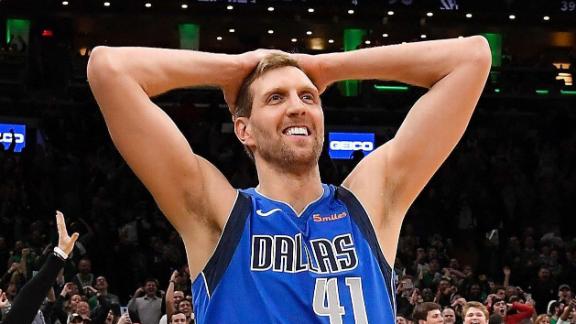The image is a vibrant photograph taken during a basketball game, capturing a player at chest level, centrally framed. The man has short, dark blonde hair with a bit of scruffy facial hair. He stands with both hands resting on top of his head, gazing towards the top right, and laughing with his teeth visible. He is wearing a bright blue jersey emblazoned with "Dallas" in black font and the number 41 in white. The jersey also features a small "5 miles" logo. Behind him, the stands are packed with cheering and happy fans. Further behind the fans, one can see the green pillars and ceiling lights of the arena, along with screens displaying advertisements.